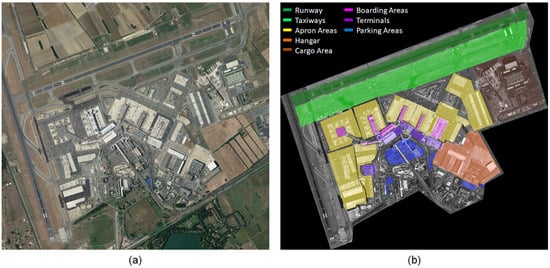Two side-by-side photos depict an aerial view of an airport complex. The left photo, labeled with an (A), shows a high overhead view of the airport, displaying numerous small, light-colored, rectangular buildings primarily situated in the lower center. The terrain includes irregularly shaped roads, brown land patches, and green grass plots in the lower corners. The right photo, labeled with a (B), presents the same airport in a more detailed and color-coded layout with a black background. This image features a titled rectangular design, with each section color-coded according to a key in the upper left corner. The key designates various areas: a green strip indicating the runway, lighter green for taxiways, orange for hangars, red for cargo areas, pink for boarding areas, purple for terminals, and blue for parking areas. This detailed, multicolored diagram clarifies the infrastructure and layout of the airport, which is less discernible in the high-altitude photo.